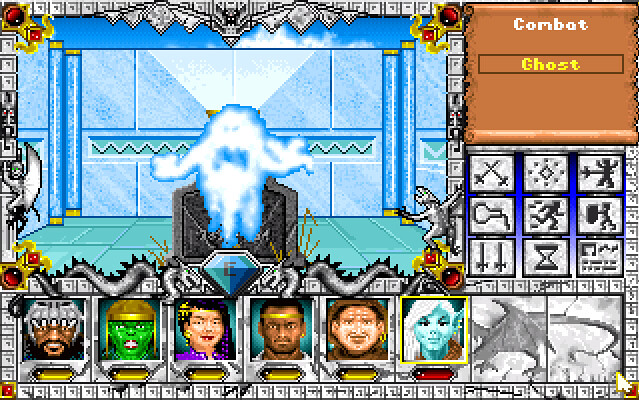This image is a detailed screenshot from a video game, showcasing a vibrant and intricate scene. The background features a gradient of cyan and dark blue, with a cyan blue wall adorned with matching pillars, set against a dark blue sky filled with white clouds. Flanking the scene are statues resembling gargoyles, positioned to the left and right atop a bluish-green tiled floor. 

The right side of the screen displays a detailed legend with various icons, enclosed in black squares: two crossing swords, a diamond with dots, a sword piercing a silhouette, a vase pouring liquid, a simple black line, a running figure with motion lines, an individual with an uplifted shield, two side-by-side swords, an hourglass, and a piece of paper with writing. Adjacent to this legend is a gray section depicting six character icons in a vertical arrangement.

Prominently in the center is a ghost, wispily outlined in lighter blue, rising above a dark gray and black cobblestone grave. The ghost features dark blue eyes, a dark blue mouth, and wispy hands, contributing to its ethereal appearance.

At the bottom, there are six character icons representing diverse avatars: 

1. An African American character with a gray wolf-like helmet.
2. A green-skinned character with pink lips and a gold helmet.
3. A character with dark purple and black hair, fair yet brown skin, pink lipstick, and a purple shirt.
4. Another African American character with black hair, a gold headband, and a gray shirt.
5. A character in a brown robe, with black hair and a golden ring in his right ear.
6. A female, elven-like character with cyan blue skin, white hair, black eyes, and wearing white attire with brown embroidery.

Finally, the top right corner of the screen includes a tan vertical rectangle with "Combat" in white font, and beneath it, a black-outlined rectangle with the yellow word "Ghost." Scattered at the corners are golden-yellow items tinged with red, adding to the scene's dynamic composition.